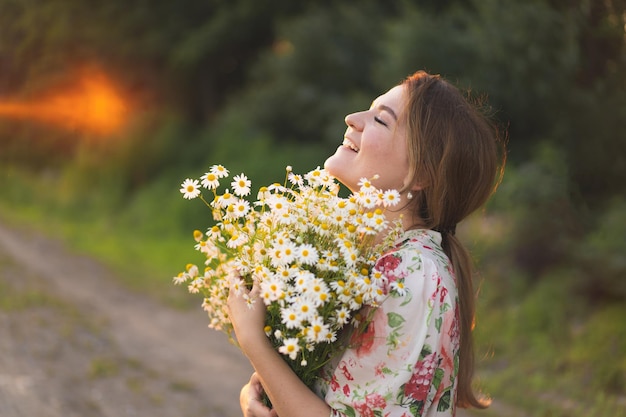In this image, a young woman is centrally positioned outdoors, illuminated by the daytime sun, which bathes her smiling face and closed eyes in a warm glow. She is seated on a concrete walkway, surrounded by lush greenery with trees and grass in the blurred background. Her long dark brown hair, styled in a mid-parted ponytail, cascades down her back. Donning a white dress adorned with dark pink flowers and light green leaves, she exudes happiness. The woman clutches a bunch of white daisies with yellow centers, holding the flower parts with her right hand and the stems with her left. She is tilting her face upwards towards the sun, with the flowers lightly touching her chin, conveying a moment of serene joy and peaceful connection with nature.